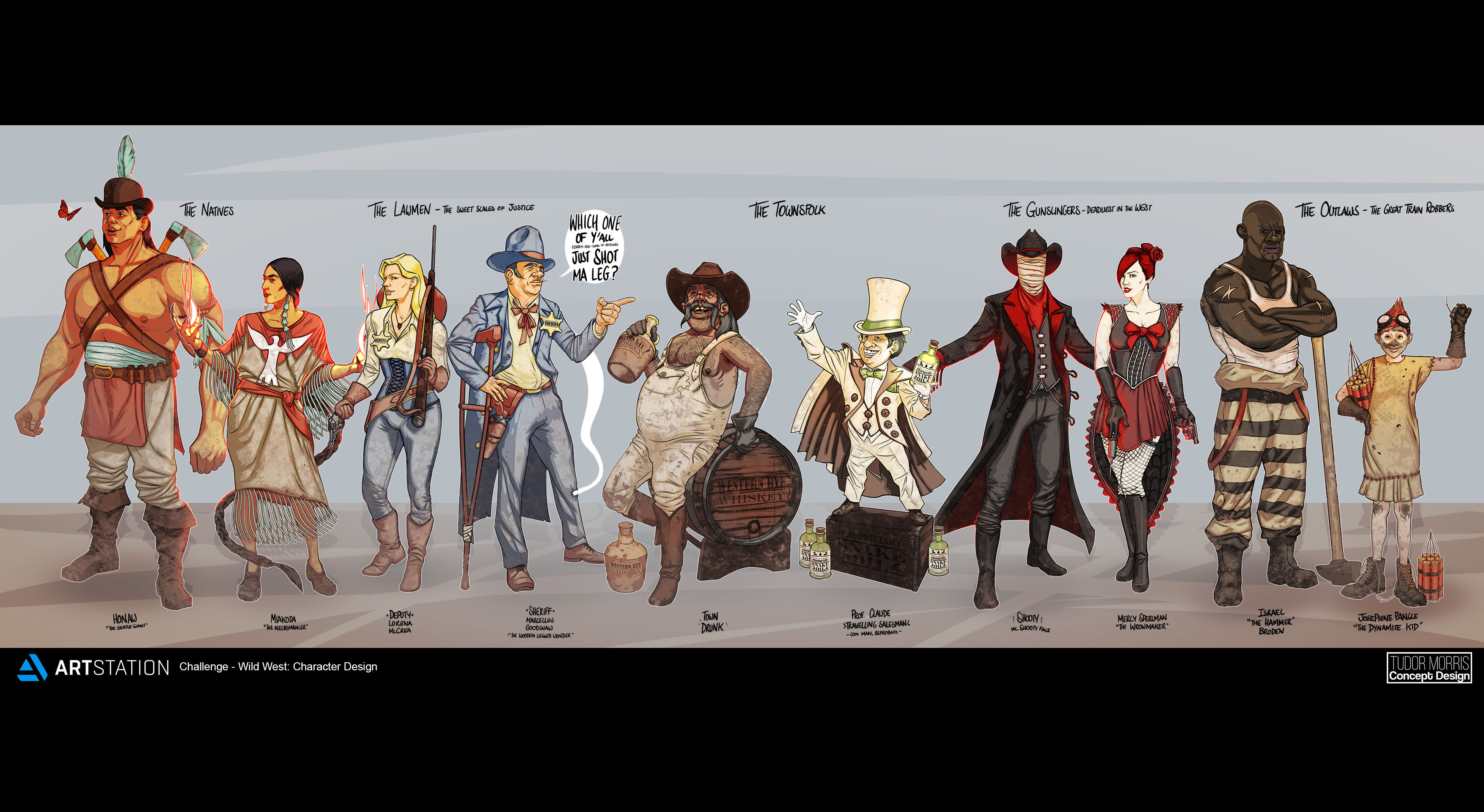This rectangular poster features a detailed lineup of diverse characters, arranged in a neat row against a colorful backdrop. A prominent black border frames the top and bottom of the image, with the bottom border displaying the Art Station logo on the left corner and another logo on the right. Each character's name is displayed above and below their images, accompanied by the author's information.

From left to right, the lineup begins with a large man resembling an Indian warrior. He wears a feathered hat, has no shirt, and dons light pants and brown boots. Two crisscross belts across his chest hold axes. Next is an Indian woman with long hair, dressed in a red shirt with a white bird emblem, holding a bag. Following her is a blonde woman with a rifle in her left hand, sporting a light-colored shirt, blue jeans, and boots.

Beside the rifle-wielding woman stands a sheriff in a light blue suit with matching hat, blue jeans, and a pistol on his belt. Continuously, a man in overalls leans against a whiskey barrel, drinking from a jug. A diminutive man, reminiscent of a midget ringmaster, stands next, clad in a white suit and top hat.

Adjacent to the small man is a cowboy with a concealed face, shrouded in bandages, wearing a long jacket and cowboy hat. Next is a showgirl with red hair, dressed in a shirt with a red bow and a red skirt. Beside her stands a muscular black man in a white tank top and prison-striped pants. The sequence concludes with a small girl in a yellow and tan dress, adorned with goggles atop her head.